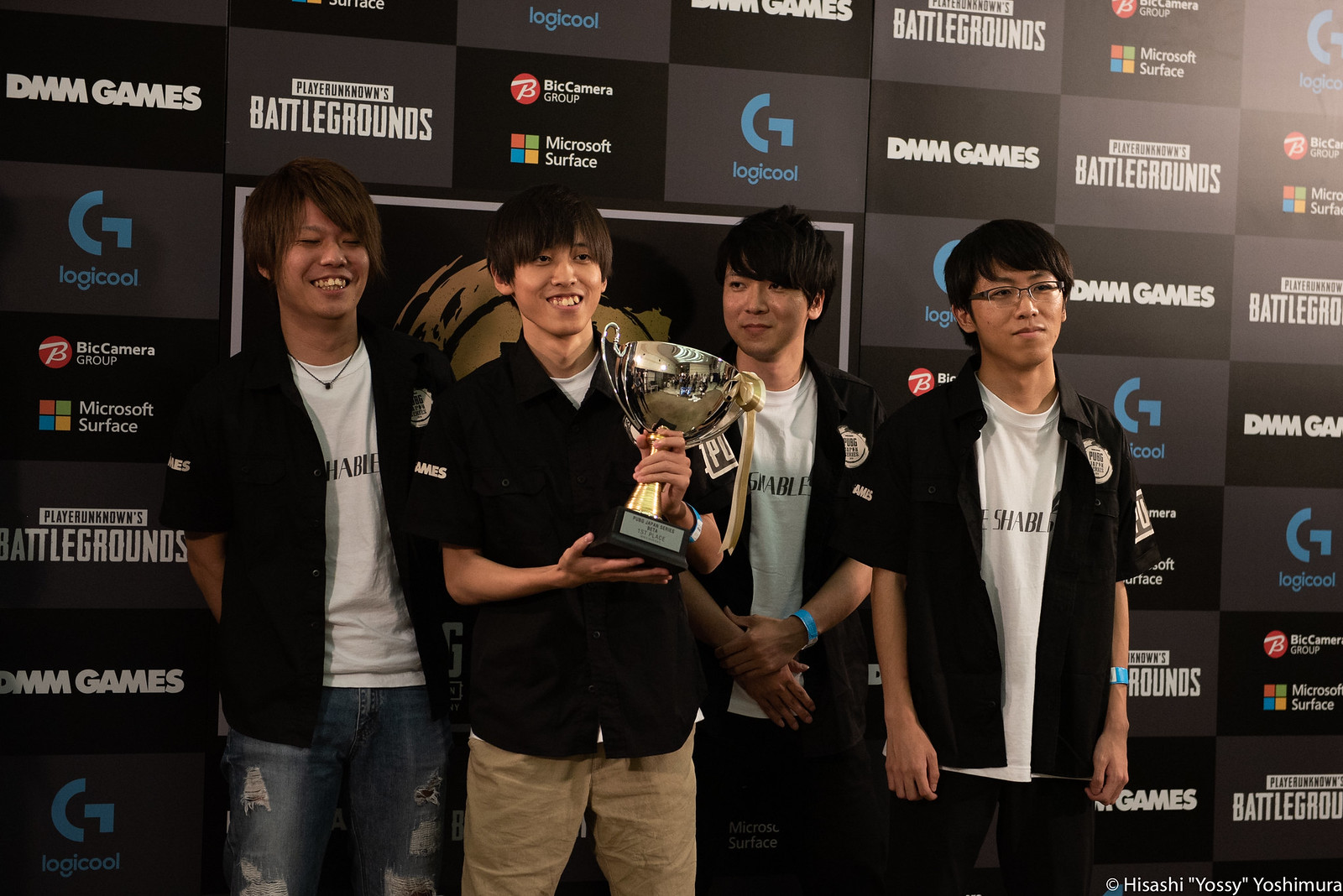In this image, four Asian teenagers stand together without posing for the camera, seemingly after winning a gaming tournament. All four wear black button-up shirts over white t-shirts, with three of them leaving their black shirts open to reveal the white shirts underneath. The white shirts have some writing on them, although the exact words are unclear. The second teenager from the left, who has black hair and is supporting a trophy with both hands, holds the cup at about chin level. The teen on the far right is adorned with glasses. Most of them have blackish hair that falls over one eye, except for the far-left teenager who has brownish hair. The background is filled with a diagonal pattern of rectangular banners featuring repetitive advertisements for brands and products such as "PlayerUnknown's Battlegrounds," "DMM Games," "Logicool," "Big Camera Group," "Microsoft Surface," and more. There’s a tag at the bottom right that reads, "© Hisashi Yassi Yashimura." The group's joyful expressions suggest their victory and the celebratory moment.